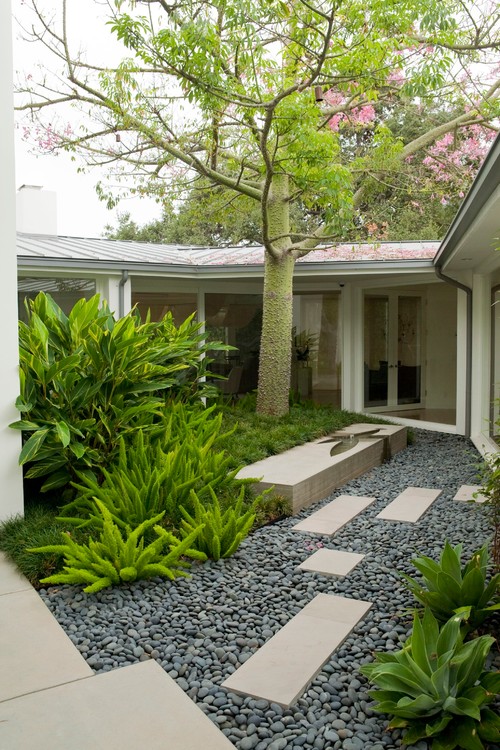This photograph captures a serene, outdoor courtyard enclosed by a single-story house with gabled roofs and walls lined with floor-to-ceiling glass windows and doors. The sky above is a hazy, whitish-gray, creating a soft backdrop for the scene. Dominating the center of the courtyard is a tall tree with a light brown trunk and lush, green foliage that towers over the house. The courtyard floor is a mosaic of dark gray crushed rocks interspersed with lighter gray concrete stepping stones, creating a contrasting patchwork. In the bottom left corner, you can see a cluster of bright green, tapered-leaf plants that add vibrant color to the setting. Additional shrubs frame the picture, particularly on the bottom right, enhancing the natural feel. A sleek, rectangular gray bench made of stone or concrete sits near the walkway, providing a minimalist seating area. The tranquil, well-designed space suggests a perfect blending of nature and architecture.